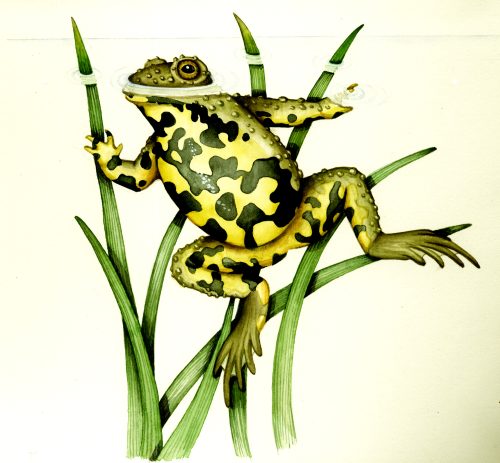The image is a detailed, square-shaped drawing of a frog partially submerged in clear, white water against a predominantly tan background that darkens towards the bottom right corner. The frog, depicted in vibrant yellow with black splotches and warts, has only its head, eyes, and one finger breaking the water's surface. The rest of its yellow and black body, including its legs spread out as if poised to kick, remains underwater. Surrounding the frog are seven blades of green grass, their stems mostly underwater while some parts extend above the surface. The frog's eyes are green, giving it a piercing look as it emerges from the water. The overall scene evokes an illustration you might find in an old textbook, with fine details on the frog's webbed feet and its scattered warts, set against the textured, shadowed background.